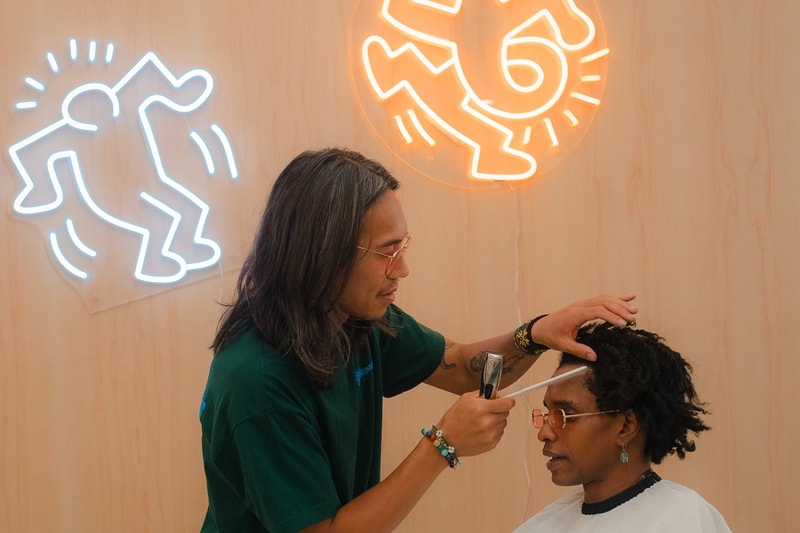In this detailed photograph of a hairstylist's salon, the backdrop features a wall with a distinct peach-colored wooden texture illuminated by two vibrant neon signs. The sign on the left displays a stylized figure dancing in blue light, while the one on the right shows another dancing outline in golden-orange light, though partially obscured. In the foreground, a hairstylist, who appears to be of Asian descent, is meticulously working on a client's hair. The hairstylist has shoulder-length salt-and-pepper hair, adorned with glasses that have rose-tinted lenses, and his arms bear intricate tattoos and multiple beaded bracelets. Dressed in a dark green t-shirt, he stands to the left, using his left hand to style the hairline with a white comb and holding a razor in his right hand. The client, sitting to the right, is draped in a traditional white barber cape and sports short, natural black dreadlocks. The client is accessorized with dangling blue earrings and pink-tinted glasses. The composition and ambiance of the salon are captured with a modern, stylish flair.